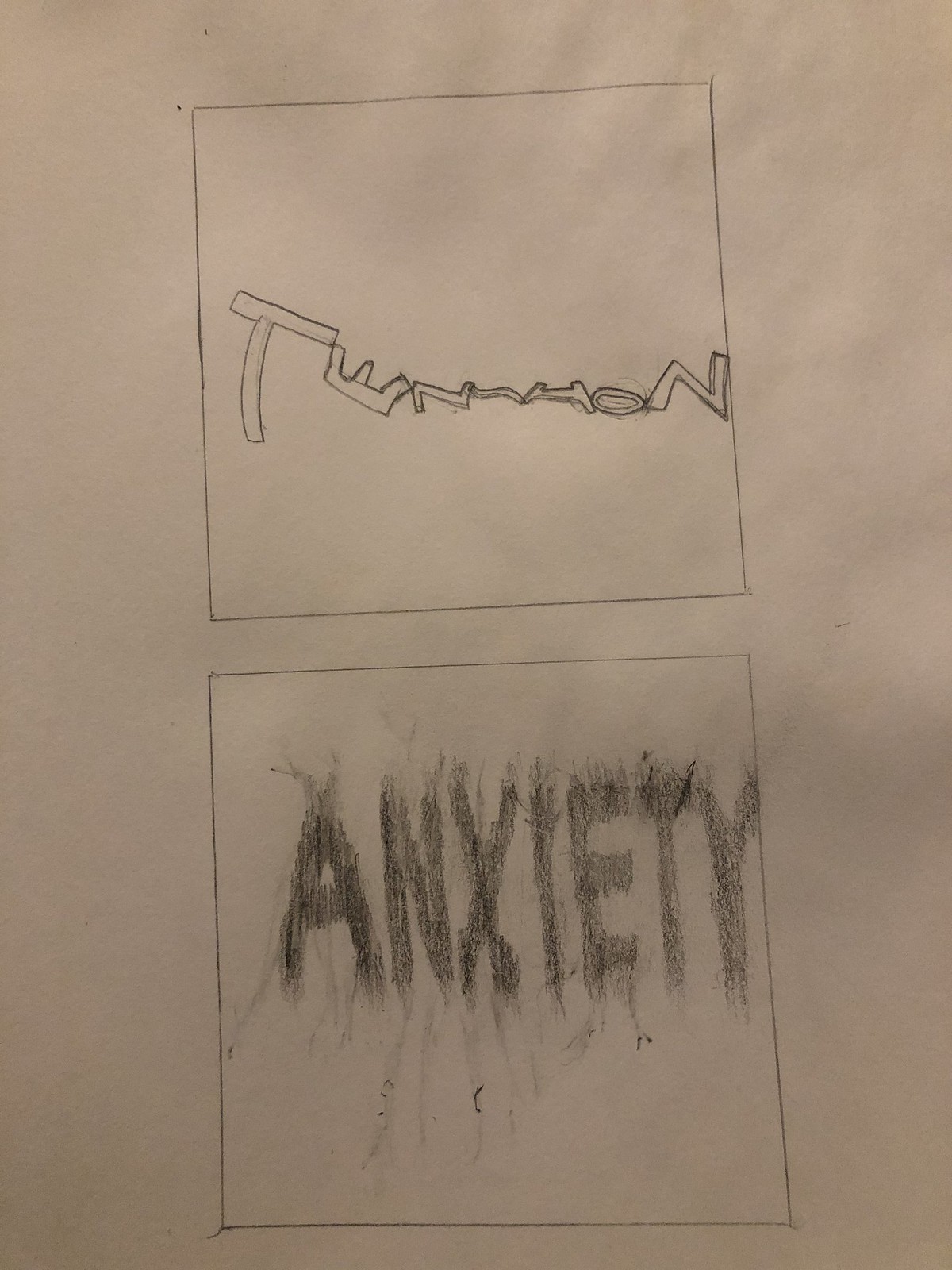This image features a hand-drawn artwork on a white piece of paper. At the upper section of the page, there is a meticulously sketched rectangular box, outlined in pencil. Inside this box, a series of letters are arranged, drawn in a whimsical, stick bubble-letter style. The letters—T, E, N, H, O, and N—rest on their sides and are scattered in a somewhat haphazard manner, making them slightly difficult to decipher at first glance.

Directly below this, there is another prominent element of the drawing: the word "ANXIETY" written in bold pencil strokes. Surrounding this word, there are dynamic, radiating lines, as if to emphasize the intense energy or emotion associated with it. The composition of the drawing carefully juxtaposes the chaotic yet contained nature of the letters in the box above with the explosive, outward movement depicted around the word "ANXIETY" below, creating a striking visual representation of emotional turmoil.